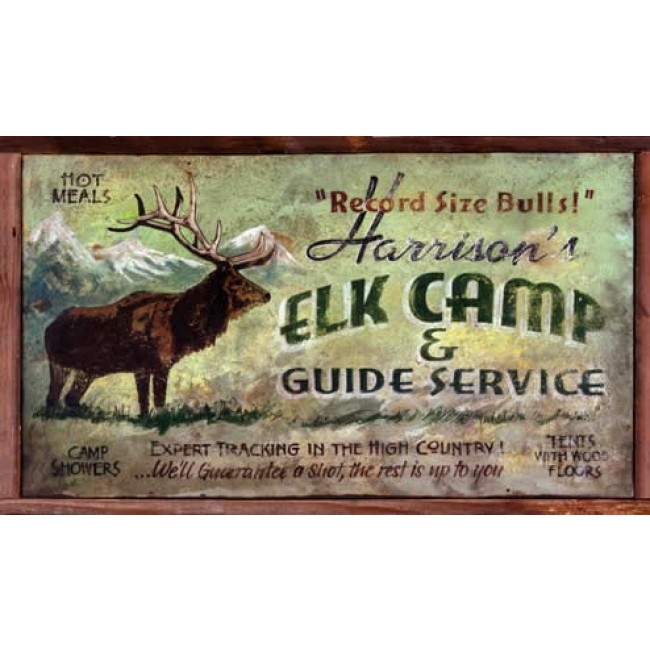The sign, with a raw wooden frame giving it a rustic, vintage feel, appears to be an advertisement for "Harrison's Elk Camp and Guide Service." The left side features a cartoonish drawing of a brown elk with large, beige antlers set against a backdrop of snow-capped mountains and patches of grass. The background of the sign has a greenish, speckled, and faded texture, enhancing its weathered charm.

Prominently displayed in various fonts, the text reads: "Record-Sized Bulls," "Harrison's Elk Camp and Guide Service," "Hot Meals," "Camp Showers," "Tents with Wood Floors," and "Expert Tracking in the High Country." At the bottom, a tagline assures, "We guarantee you the shot, the rest is up to you." The overall layout blends bold green letters and relaxed cursive script, emphasizing the guide service's offerings and commitment to a successful hunting experience.